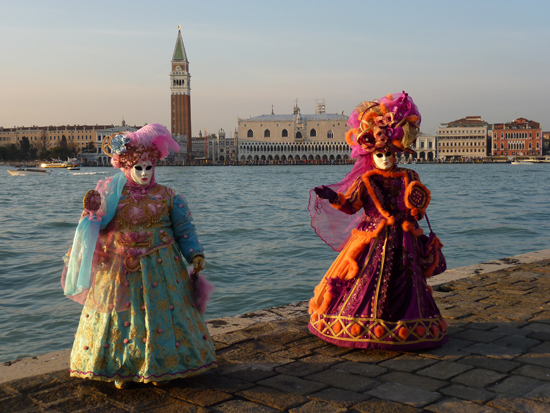The image features a striking and detailed cityscape set against a gray and bluish-white sky. Horizontally spanning the background, an array of buildings dominates the scene. On the left and center are long, whitish-tan structures, with a prominent tall, slender building featuring a steeple nestled between them. To the right, shorter buildings in white and red add diversity to the skyline. The entire cityscape is bordered by a body of water, enclosed by a constructed wall.

In the foreground, two women stand near the water's edge. Positioned slightly left and right of center, one stands further back than the other. They are dressed in elaborate, poofy dresses that flare out at the bottom, each adorned with distinctive headdresses. The woman on the left wears a bluish outfit with a headdress reminiscent of cotton candy, while the woman on the right is dressed in an orange-red ensemble with a floral headpiece. Both women don masks and feathered accessories, exuding an air of opulence with their mesh capes flowing behind them. The attire evokes a traditional, perhaps geisha-inspired aesthetic, adding a vivid cultural flair to the already rich scenery.